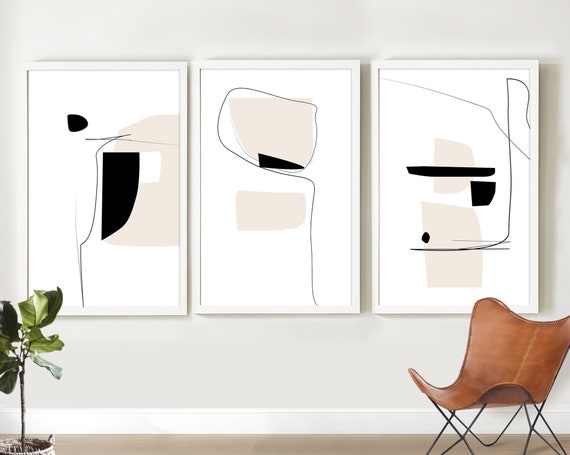The image is taken indoors and showcases three evenly spaced rectangular paintings, all created in an abstract, graphic art style by the same artist. Each painting features a white background adorned with peach or light pink splotches and irregular black shapes. The leftmost painting has a central peach shape overlain by a large black blotch, a smaller black spot in the top left, and a thin, sketched black line. The middle painting contains two peach splotches, a near-triangular black shape, and a similar thin black line. The painting on the right includes two peach splotches, a central horizontal black line, a square black blotch below and to the right, and another black shape towards the bottom left with the same kind of thin line. Below these paintings, the room features a floor with a brown color and white trim at the wall edges. A brown metal-framed chair is positioned to the right, and a green plant with a long stem in a white pot is placed to the left, likely artificial.